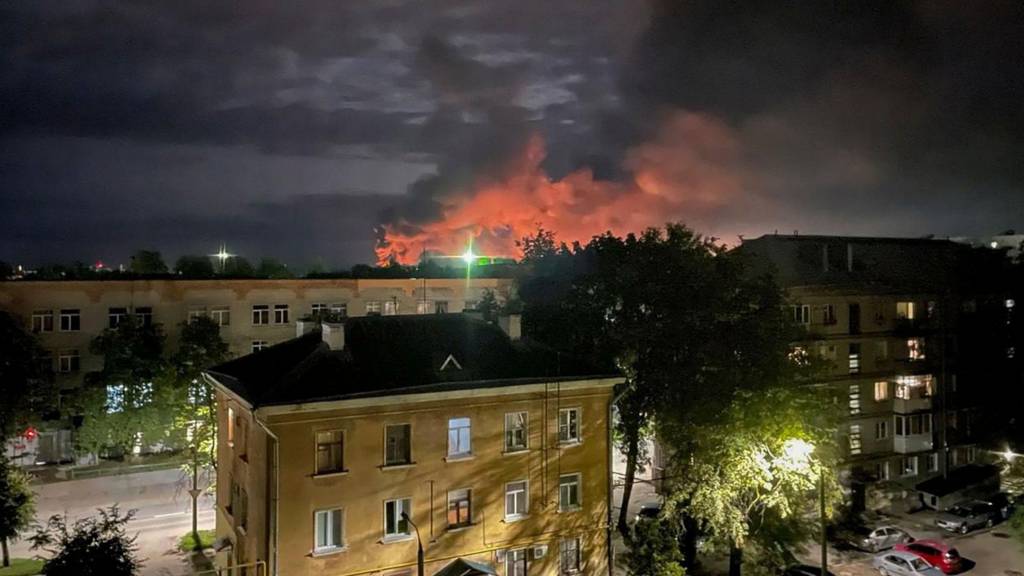This color photograph, taken at night, captures a cityscape from perhaps a rooftop or balcony perspective. In the foreground, two residential buildings, likely apartment complexes, stand prominently. The central building is brown with a black roof and white window frames, spanning approximately three stories. Adjacent to it on the right is a shadowed building, also brown with a dark gray roof. Between these structures are two tall trees illuminated faintly by a nearby streetlight, and a parking lot with four cars—three silver and one red—can be seen in front of them. Another separate apartment building is visible beyond this parking area. A wide street runs horizontally across the scene, separating the foreground buildings from the distant ones. In the background, there is a long rectangular building with a gray facade and a brown top, featuring many white-framed windows. Above all this, the night sky extends across the horizon, mostly dark with slight illumination from distant city lights. Dominating this nocturnal backdrop is a dramatic display of thick, reddish clouds billowing up, suggesting a possible fire or explosion, adding an ominous yet captivating element to the night scene.